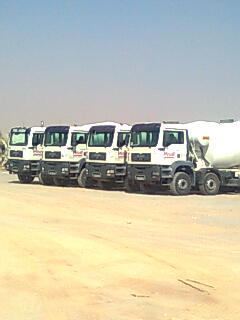This is an image of four heavy industrial trucks, likely cement mixers, parked close to one another in a sandy, desert-like area. Each truck features a large, boxy white cab with black trim around the windows and black front bumpers. The vehicles are predominantly white with some indiscernible red text or logos on the doors. The trucks are positioned side by side, facing slightly left, which gives a view of their front and side profiles. Behind the cabs, there is a visible cylindrical compartment typical of cement mixers. The trucks also have large black tires with silver rims, emphasizing their robust design. The ground is a yellowish-tan, sand-colored terrain, and the sky above is clear with a gradient from pinkish-blue at the horizon to a lighter blue higher up. The overall setting suggests a hot, arid environment with no clouds in sight, indicating it's daytime.